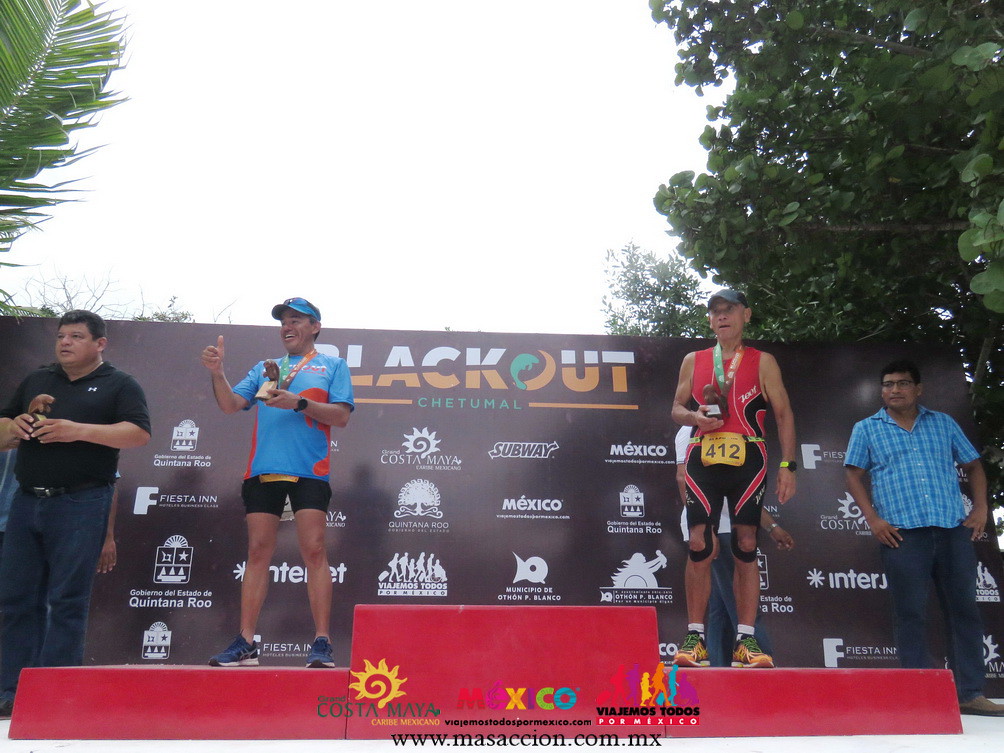This photograph captures the aftermath of a marathon held in Chetumal, prominently featuring the winner's stage adorned by four men. Dominating the backdrop is a display board reading "Blackout Chetumal" in green, accompanied by sponsor logos from various companies like Subway and Municipio de Othon P. Blanco. 

On the far left stands a man in a black polo shirt and blue jeans, holding a brown item in his hands. Just to his right, another man in a blue shirt, black shorts, blue cap, and blue sneakers is giving a thumbs up while holding a brown and gold trophy. 

In the center, the highest step of the winner's podium is notably empty. Moving to the right, a participant in a red tank top with the number 412 prominently displayed, yellow racing pants, and a gray and black cap holds a small trophy and wears a medal around his neck. 

Finally, on the far right is a man in a blue collared shirt, blue jeans, and glasses. They all stand beneath a clear white sky with the shadow of a tree visible above them, encapsulating the celebratory atmosphere of the event.